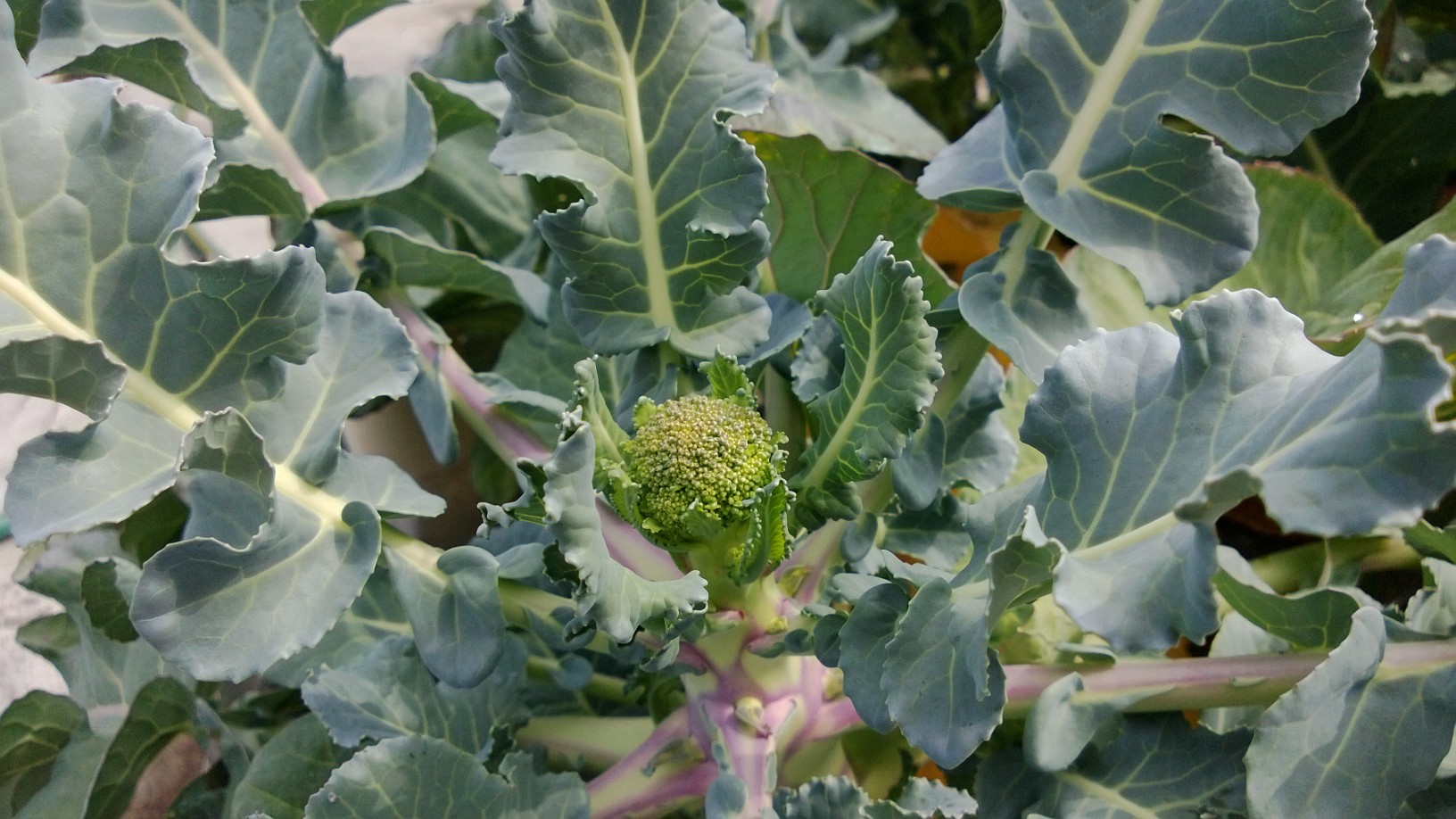This color photograph showcases an edible plant that appears to be a form of leafy greens, possibly collard greens, sprouting in a manner reminiscent of a flower. Central to the image is a small bundle that bears a resemblance to the head of a broccoli, both in its green coloration and textured appearance. The leaves, forming the bulk of the composition, radiate outward in a rosette pattern. These leaves are predominantly a rich green with light green veins coursing through them, lending a vivid contrast. Some leaves exhibit shades of greenish-blue, with crinkled and ridged textures along the edges. The stems and stalks, visible beneath the leaves, present a mix of whitish and light green hues, interspersed with pinkish-purple veining. Additionally, there are smaller, younger leaves clustered around the base of the plant. The detailed leaves range from six inches to longer, filling the entirety of the photograph and obscuring any background. Shadows cast by the leaves introduce darker crevices at the top right, adding depth to this vibrant, intricate portrayal of the leafy plant.